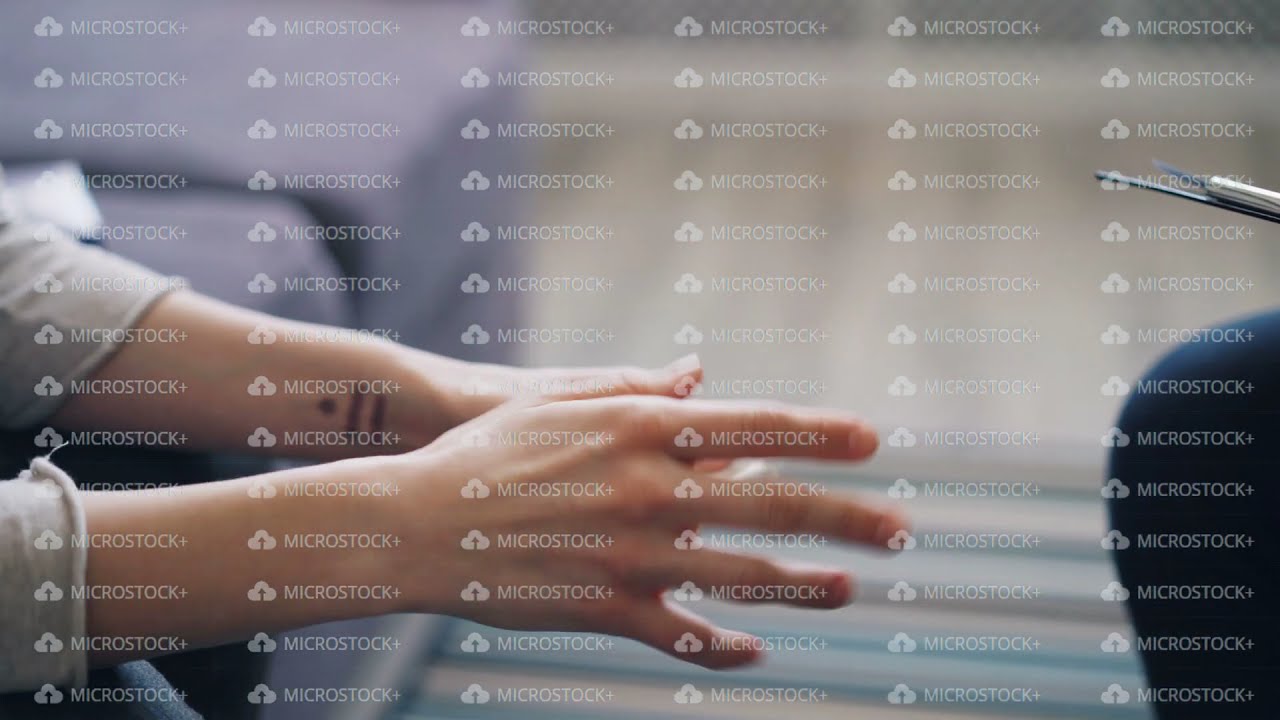In this stock photo, a woman’s hands, clad in a gray-sleeved shirt that stops mid-forearm, extend from the left towards the center of the image, revealing a small tattoo on her left wrist. The background is blurred but shows a gray couch against which she sits, and the floor appears white. On the right side of the image, a person’s knee in jeans is visible, along with what seems to be a notepad or clipboard they are holding. The background transitions in color from gray on the left, to beige and green on the right, with a blue chair back partially visible. The entire image is overlaid with numerous watermarks reading "Microstock Plus" alongside a logo of a cloud with an upward arrow, emphasizing its nature as a stock photo.